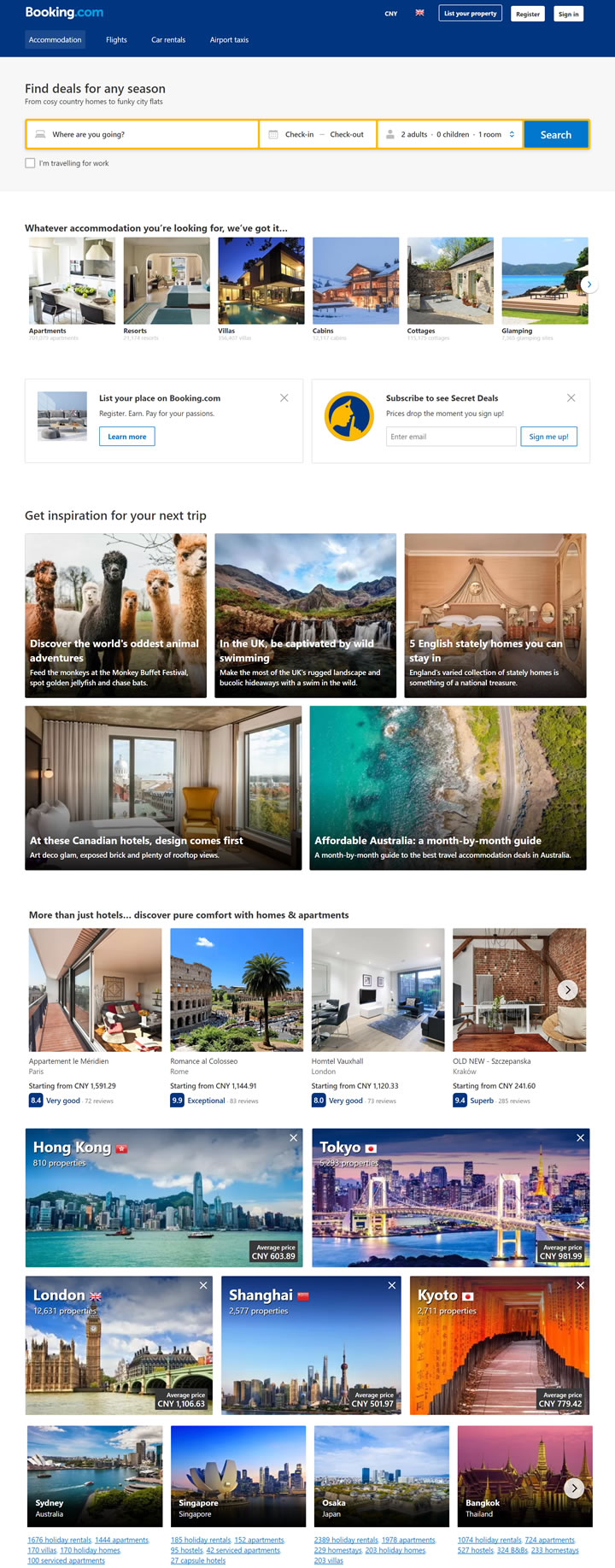### Booking.com Website Homepage Overview

**Header:**
- **Logo:** The "Booking" text is in white, while ".com" is highlighted in blue, all set against a navy banner.
- **Navigation Menu (Left to Right):**
  - **Accommodation**
  - **Flights**
  - **Car Rentals**
  - **Airport Taxis**
- **Action Items (Right Side):**
  - "List your property" in a white banner.
  - "Register" and "Sign In" in white banners.
  - Currency indicator “CYN” with a UK flag.

**Main Content:**

- **Search Section:**
  - Background Color: Gray.
  - Tagline: "Find deals any season, from cozy country homes to funky city flats."
  - **Search Banners (Outlined in Yellow):**
    - "Where are you going?"
    - "Check in"
    - "Check out"
    - Dropdowns: Number of Adults, Children, Rooms.
  - **Search Button:** Blue with white text "Search."
  - **Optional Checkbox:** "Traveling for work?"
- **Accommodation Types:**
  - **Section Title:** "Whatever accommodation you're looking for, we've got it."
  - Categories:
    - **Apartments:** Visual of a stylish apartment.
    - **Resorts:** Image of a lavish hotel room.
    - **Villas:** Visual representation.
    - **Cabins:** Scenes of mountain cabins with snow.
    - **Cottages:** Picture of a quaint cottage.
    - **Glamping:** Image of a hut over turquoise waters with a chaise lounge.

**Promotional Offers:**
- **Listing Incentive:** Blue banner stating "List your place on Booking.com" with "Learn more" in blue text.
- **Subscription Box:** "Subscribe to see secret deals" with an input for email addresses.

**Travel Inspiration:**
- **Article Titles and Images:**
  - "Discover the world’s oddest animal adventures" with alpacas.
  - "Be captivated by wild swimming" in the UK, showing mountains and waterfalls.
  - "Five English stately homes you can stay in" illustrated with a luxurious bedroom.
  - "At these Canadian hotels, design comes first," showcasing trendy interiors.
  - "Affordable Australia: month by month guide" depicting a beach with turquoise water.

**Additional Recommendations:**
- **Headline:** "More than just hotels, discover pure comfort with homes and apartments."
- Example Listings:
  - **Apartment in Meridian, Paris**
  - **Romance at Colosseo, Rome**
  - **Hometown, Vauxhall, London**
  - **Old, New, Satchipacha, Krakow**
  - Each listing includes starting price and ratings.

**City Guides:**
- Featured Cities:
  - Hong Kong
  - Tokyo
  - London
  - Shanghai
  - Kyoto
  - Sydney
  - Singapore
  - Osaka
  - Bangkok
- Each city entry includes:
  - Image of the city
  - Map icon and flag
  - Average price in CNY
  - Count of accommodation options like hotel rentals, apartments, villas, holiday homes, and serviced apartments.

**Footer:**
- Detailed accommodation statistics for each featured city such as:
  - 1,676 hotel rentals
  - 1,444 apartments
  - 170 villas
  - 170 holiday homes
  - 100 serviced apartments

This comprehensive breakdown offers a detailed snapshot of the Booking.com homepage, helping users navigate through various booking options, travel inspirations, and accommodation types efficiently.